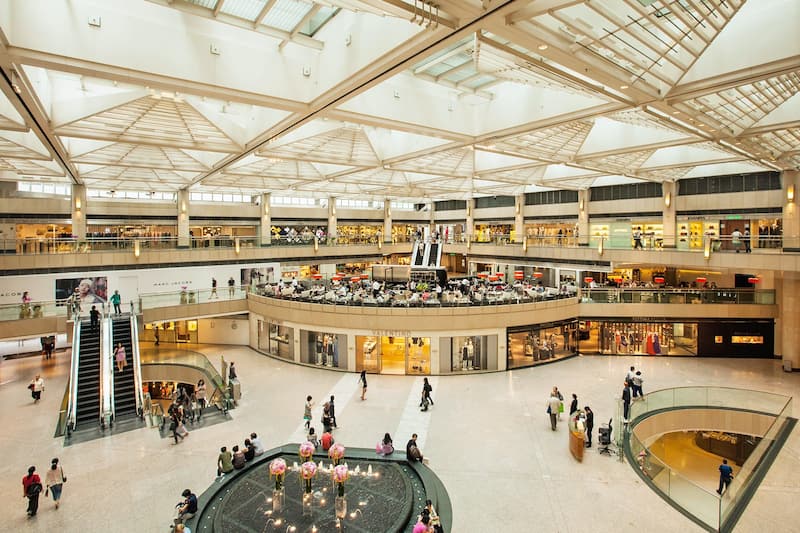The image captures a bustling multi-story shopping mall from a high vantage point, revealing a dynamic and vibrant indoor scene. The view encompasses a spacious central atrium filled with people walking around on white floors. A prominent feature of the atrium is a decorative water fountain surrounded by a ledge where several people are seated. On the left side, an escalator transports people between the levels of the mall. The mall features multiple floors, each lined with various stores, and there's a noteworthy round shop centrally located, serving as a focal point of the open area. Skylights and large windows in the unique geometric ceiling flood the space with natural light, creating a bright and inviting atmosphere. The floor below the main floor is visible through a cutout with a glass railing, adding to the airy and open feel of the space. The entire setting is animated with shoppers and visitors, illustrating a lively commercial hub.